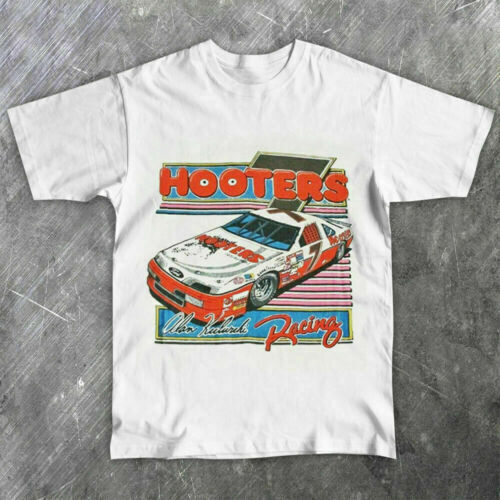The image features a white, short-sleeved crew neck t-shirt against a solid gray background with white diagonal slashes. Prominently displayed on the front of the t-shirt are the bold red words "Hooters Racing," with the 'O's designed to resemble eyes with white and black dots. Below the text are decorative stripes in shades of light blue, gray, light orange, and red. At the center of the t-shirt, there is a detailed illustration of a white race car with an orange undercarriage, bumpers, and door. The race car sports a large number 7 in black on its side, and also on top, along with multiple sponsor stickers. The hood of the car features the word "Hooters" along with the recognizable Hooters owl mascot. A light blue stripe on the car contains the name "Allen Colerick" and the word "Racing" in cursive red lettering. All these elements highlight the t-shirt's retro design, blending various colors and motifs with the racing theme.